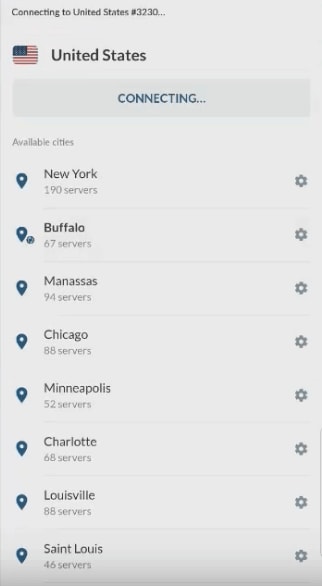The image is a screenshot from a mobile phone interface displaying connection options to various servers in the United States. In the upper-left corner, the screen reads "Connecting to United States number 3230..." with an accompanying American flag icon next to the text "United States." Beneath this, the status "Connecting" is prominently displayed.

Below the connection status is a well-organized list of available cities, each accompanied by a pinpoint icon on the left and a settings icon on the right. The list of cities and their respective server counts are as follows:

1. New York - 190 servers
2. Buffalo - 67 servers
3. Manassas - 94 servers
4. Chicago - 88 servers
5. Minneapolis - 52 servers
6. Charlotte - 68 servers
7. Louisville - 88 servers
8. St. Louis - 46 servers

The entire screenshot is rectangular in shape and features a light gray background, providing a clean and straightforward user interface layout.